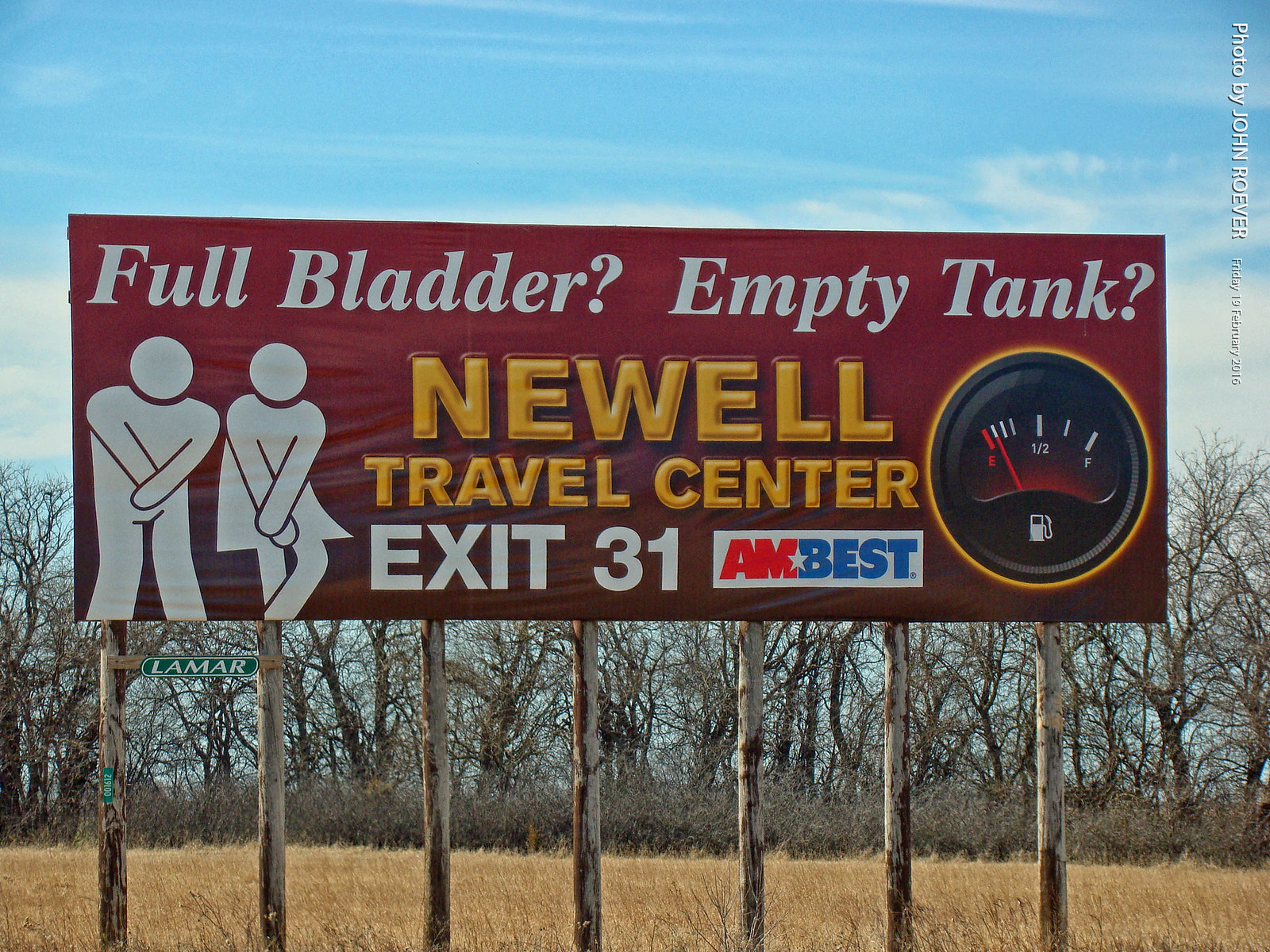This close-up photograph features a prominent, rectangular sign set against a vibrant reddish-maroon background. At the top of the sign, bold white text reads, "FULL LADDER?" followed by "EMPTY TANK?" Below these phrases, the name "NEWELL" appears in large, eye-catching yellow-orange capital letters. Beneath "NEWELL," the phrase "TRAVEL CENTER" is printed in white, and directly under that, "EXIT 31" is also displayed in white. Adjacent to "EXIT 31," there's a small white rectangle containing the letters "AM" in orange.

Central to the sign is a filled-in red star, positioned off-center, with the word "BEST" written in blue nearby. To the right, a black circle outlined in orange depicts a nearly empty gas tank. On the left side of the sign, a man and a woman are illustrated with white circular heads and filled-in bodies, slightly leaning forward with their hands crossed in front of them.

The sign is supported by narrow tree trunk posts extending from the bottom and is situated in a field of tall, wheat-colored grass. Behind the sign, there is a dense row of leafy trees, and the background is completed with a clear blue sky dotted with fluffy white clouds.